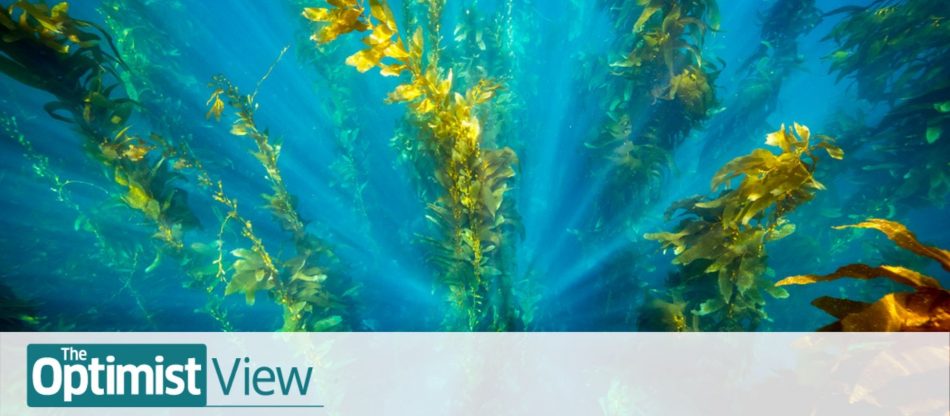The image is a rectangular underwater scene, likely a drawing, measuring approximately six inches wide by three inches tall. It showcases a vibrant blue underwater environment, dotted with light beams emanating from the center and spreading outward. 

In the foreground, tall strands of green kelp dominate the scene, with some strands fading to a yellow-gold hue as they approach the top. The kelp appears to envelop us, suggesting a dense kelp forest, though many of the plants are cut off by the edges of the image. The upper left-hand corner features a vague, fish-like shape, adding to the underwater ambiance. In the lower right-hand corner, we see detailed fawns of a kelp plant up close.

A semi-transparent gray footer spans the bottom of the image, measuring about three-quarters of an inch high. On the left-hand side of this footer, a blue-green rectangle with white print reads "The Optimist," followed by the word "View" in blue-green print, which is underlined. The overall design suggests it could be used as a heading for a website or magazine, with clear, distinct colors aimed at standing out against the vivid underwater backdrop.